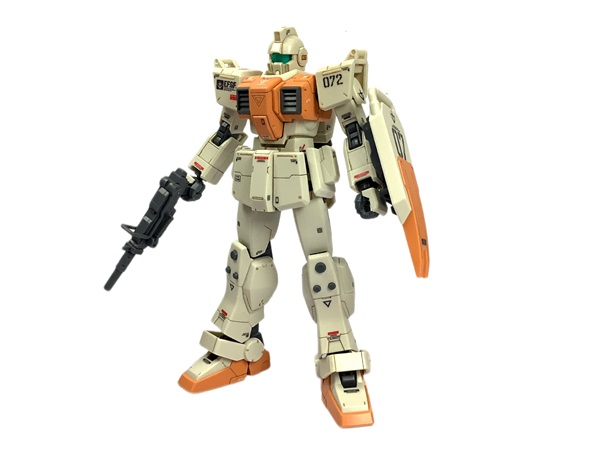The image features a detailed action figure that appears to be a Transformer or a Gundam-style robot, standing centrally against a plain white background. The action figure stands vertically and is primarily white, with patches of golden brown and orange detailing. It has a green visor on its head. The figure’s legs are white with shoes featuring white tops and brown outer soles. The torso is white at the bottom and transitions to golden brown at the top. This action figure is equipped with two arms: the left arm holds a shield accented with orange and marked with the number "707,” while the right arm is holding a long black gun and has the number "072" inscribed on the shoulder. Despite the varied color palette of gray, green, black, orange, and red, the overall scene remains stark with no other objects visible, contributing to a minimalist but detailed portrayal of the robot.